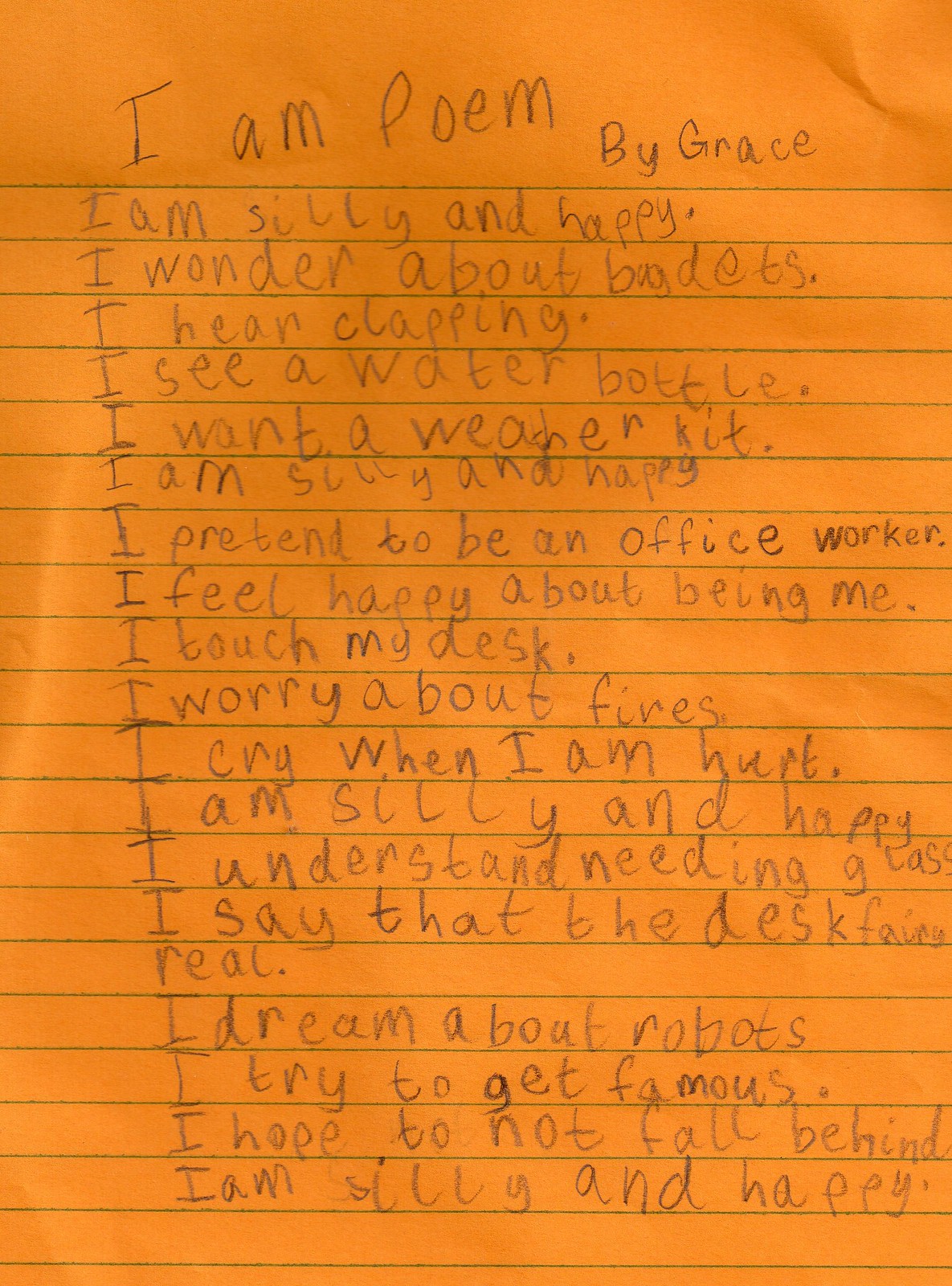The image depicts a piece of paper that appears to be from a child's notebook or journal, filled with lines and handwritten in pencil, suggesting it possibly came from a child's notebook or journal. The title at the top reads, "I am poem by Grace." The poem is written with a distinct, childish handwriting, making some parts a bit hard to read. The poem goes as follows: 

"I am silly and happy.  
I wonder about budgets.  
I hear clapping.  
I see a water bottle.  
I want a weather kit.  
I am silly and happy.  
I pretend to be an office worker.  
I feel happy about being me.  
I touch my desk.  
I worry about fires.  
I cry when I am hurt.  
I am silly and happy.  
I understand needing glasses.  
I say that the desk fairy is real.  
I dream about robots.  
I try to get famous.  
I hope to not fall behind.  
I am silly and happy."

The text, created by a young child, reflects a mix of whimsical and everyday concerns, capturing the essence of a child’s imaginative world and emotional state. The orange-hued paper adds to the warm and playful nature of the poem.